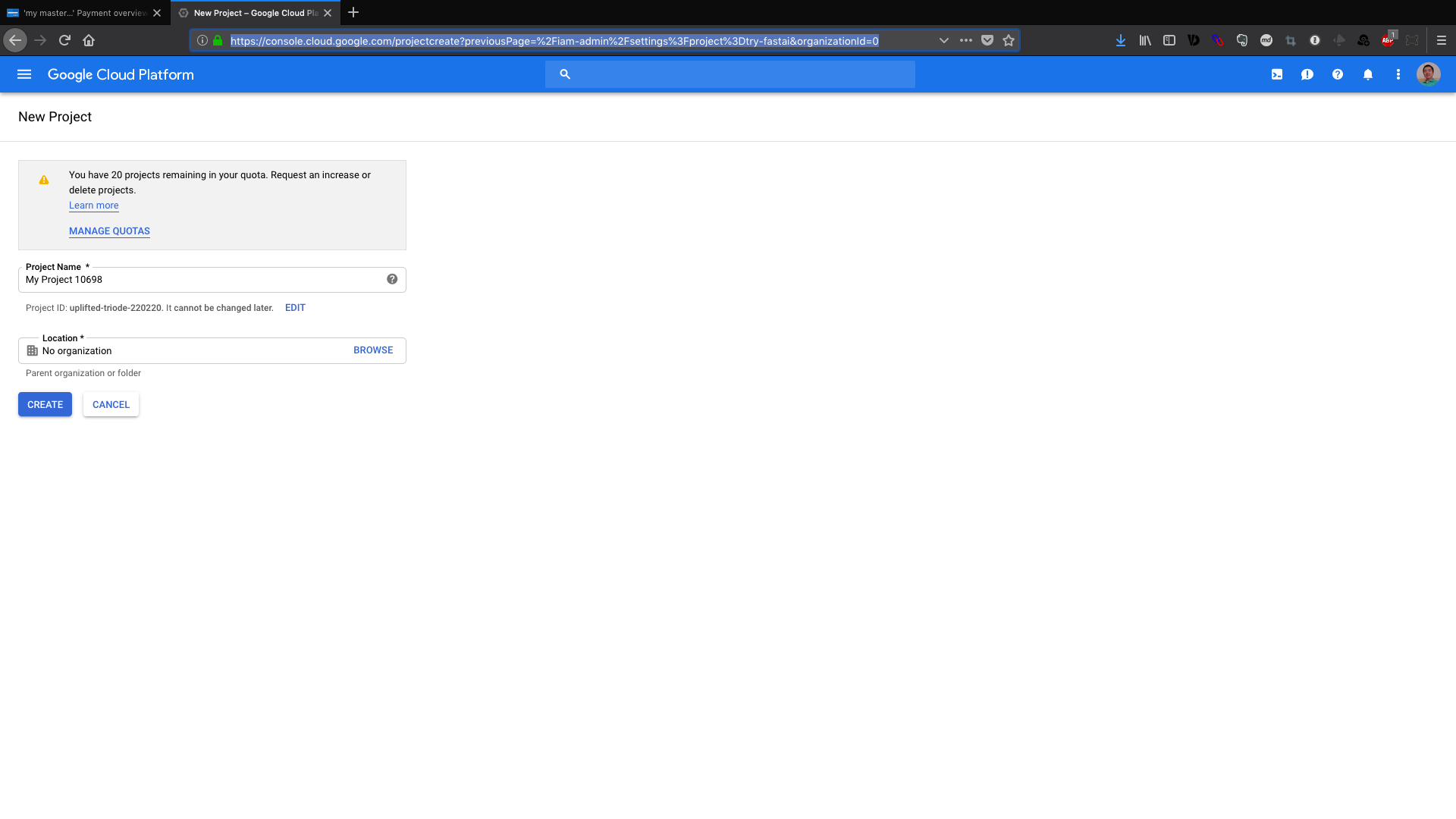The screenshot depicts a computer screen in landscape mode, likely from a laptop or desktop, showcasing the Google Cloud Platform interface. At the top of the screen, there are two open browser tabs visible on a black navigation bar, with a dark gray URL bar beneath it containing various icons on both the left and right sides.

Directly below this is a light blue navigation bar stretching across the screen. On the left side of this bar, it displays "Google Cloud Platform" next to a menu button, and in the center, a search icon is present. On the right side of the bar, there are icons, including a notification bell and a user profile with a drop-down menu. 

Below the blue bar, a light gray box informs the user that they have "20 projects remaining in your quota," with links to "request an increase" or "decline projects." This section also includes two buttons: "Learn more" and "Manage quotas."

Following this informational section, a form for creating a new project is partially visible. The form fields include "Project name" (with a default entry "My Project 1698"), "Project ID" (indistinct due to small text size), "Location" (currently set to "No organization"), and a "Browse" button situated to the left. At the bottom of this form, there are two buttons: a prominent blue "Create" button and a smaller white button labeled "Kids."

Overall, the screenshot provides a clear glimpse into the setup process for initiating a new project within the Google Cloud Platform, complete with detailed navigation and actionable options for project and quota management.